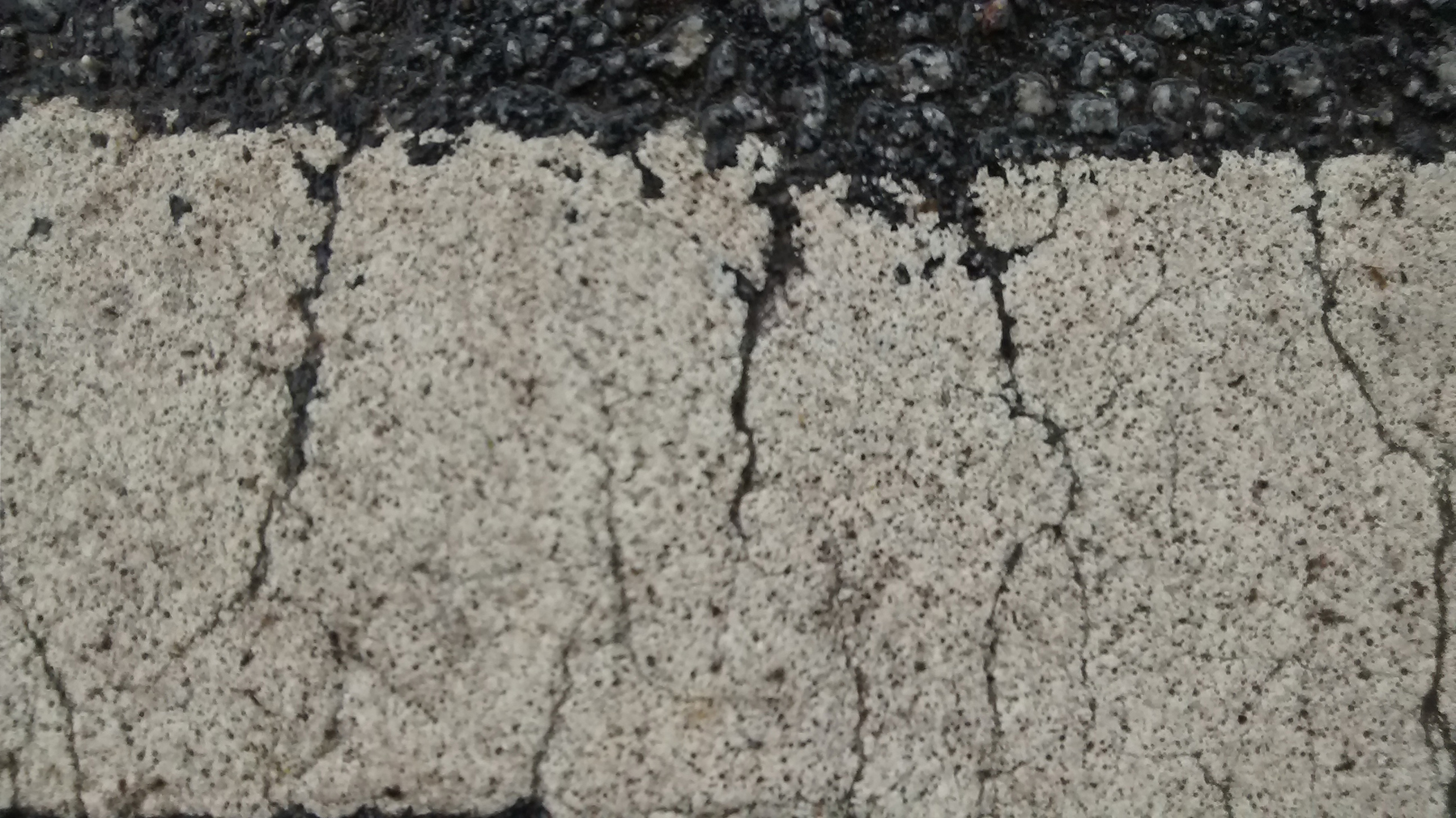This image captures a close-up view of a fragmented asphalt ground, divided into two distinct sections. The upper portion is dominated by a narrow strip featuring a mixture of loose stones, concrete fragments, and varying colors, primarily black. This top area appears heavily weathered, with evidence of the concrete disintegration into smaller pieces contributing to the scattered stones.

The bottom section of the image reveals more details of the ground, characterized by an extensively cracked concrete surface, accentuated by white paint. The paint is notably worn, with three prominent cracks slicing through it – one on the left, one in the center, and one to the right. Specks of black are visible through these cracks, hinting at the asphalt base below. Additionally, the weathered white paint is interspersed with patches where the underlying typical asphalt color is exposed, further attesting to the surface's deteriorated state.